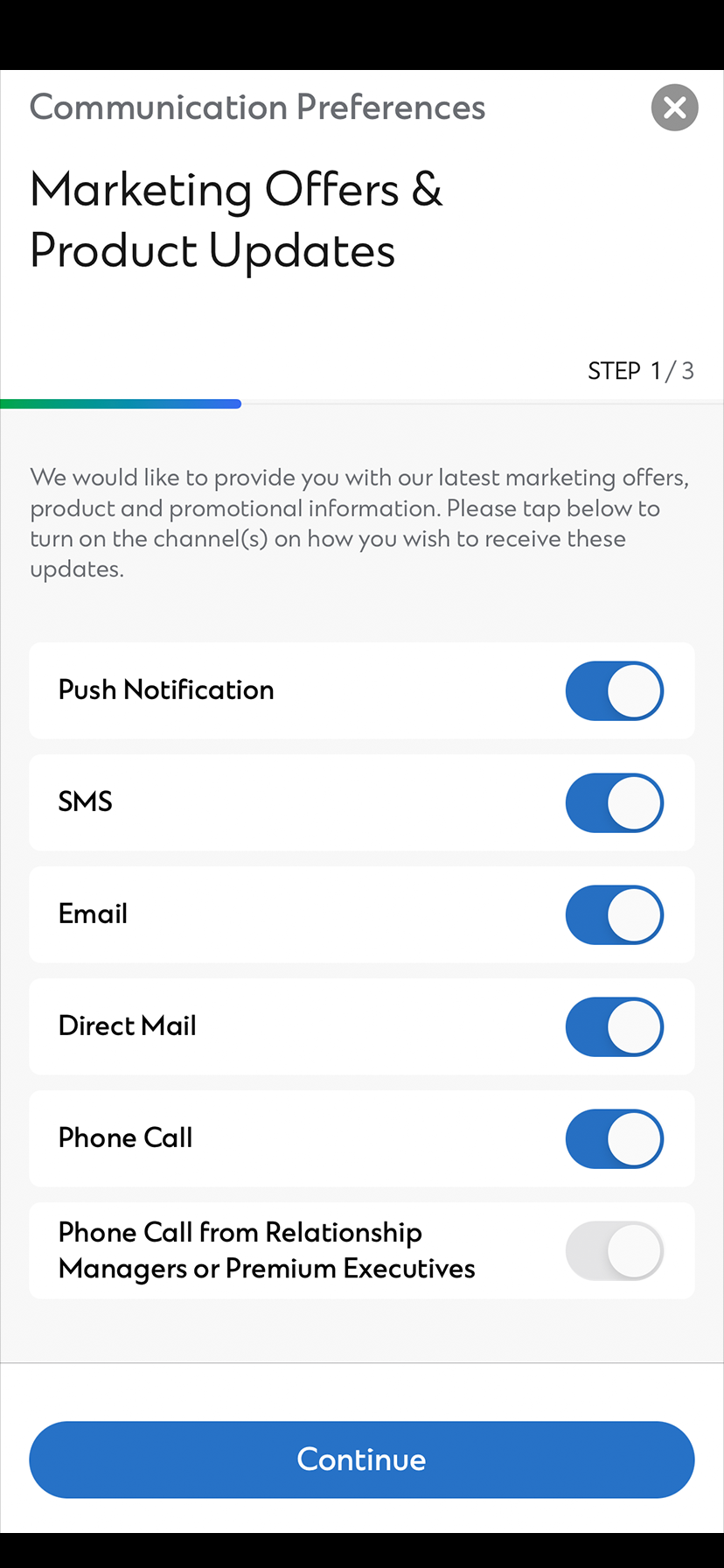The image is a screenshot taken from a mobile phone, showcasing a section of a settings page dedicated to communication preferences. The page displays several toggle options under the category "Marketing Offers and Product Updates," which encompass preferences for how the user would like to receive promotional information and updates. A brief introductory description at the top reads: "We would like to provide you with our latest marketing offers, products, and promotional information. Please tap below to turn on the channels on how you wish to receive these updates." 

The available toggle categories include:
1. Push Notification
2. SMS
3. Email
4. Direct Mail
5. Phone Call
6. Phone Call from Relationship Managers or Premium Executives

All options are currently toggled on, indicated by blue switches, except for "Phone Call from Relationship Managers or Premium Executives," which remains switched off. Beneath these options is a blue "Continue" button to advance to the next step. The screenshot features black border banners at both the top and bottom edges, framing the central content. This is the first step in a multi-step process, as indicated near the top of the page.